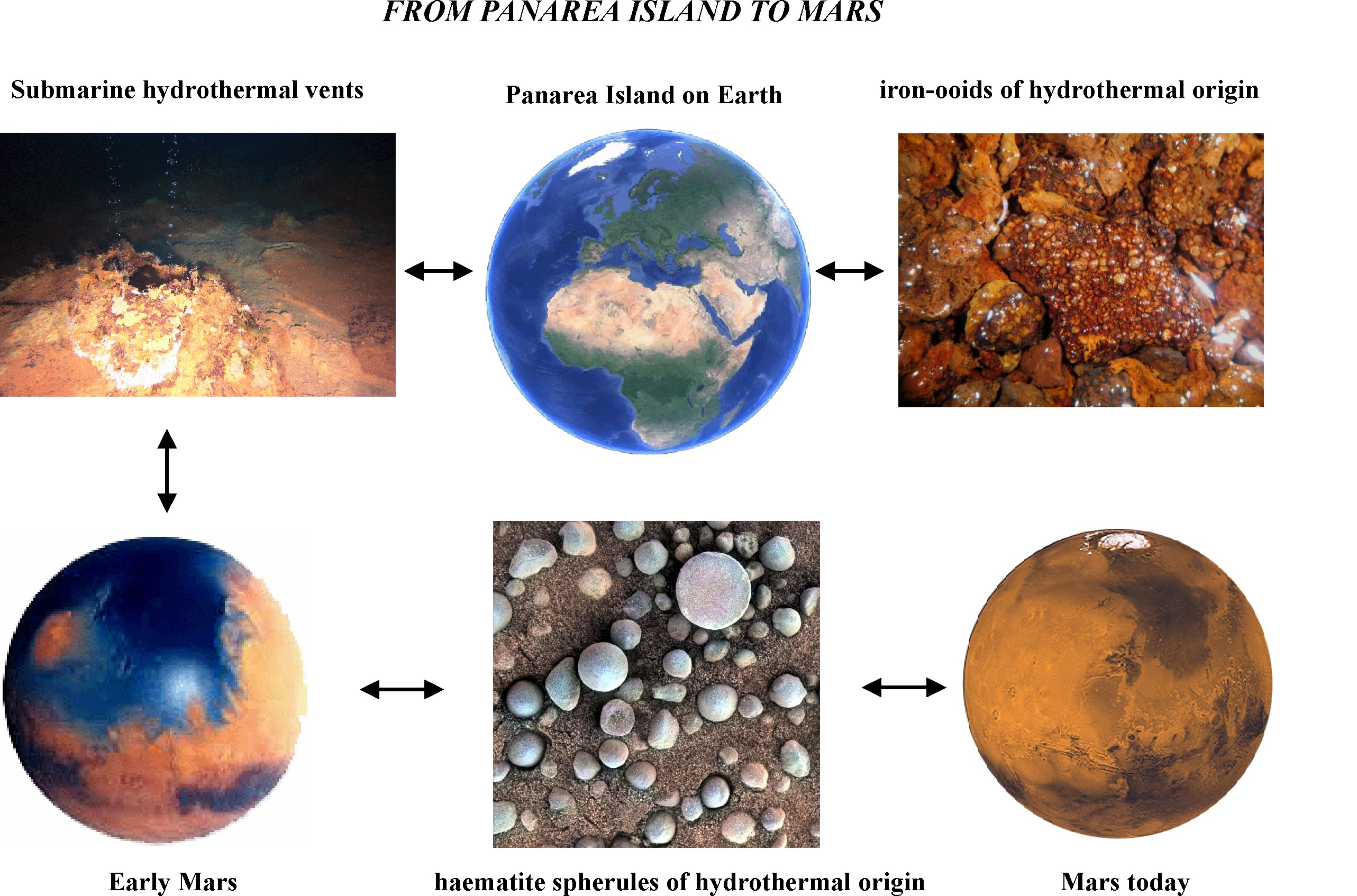This detailed scientific diagram, titled "From Panaria Island to Mars," comprises of two rows with six interconnected images. The top row begins with an image labeled "Submarine Hydrothermal Vents," depicting underwater vents with bubbles rising from them. Arrows point to the next image, "Panaria Island on Earth," showing a section of the Earth highlighting Africa, Europe, and the British Isles. An adjacent image labeled "Iron Ooids of Hydrothermal Origin" displays orange and red spherical rocks, indicating a hydrothermal origin.

The bottom row starts with "Early Mars," illustrating a planet with extensive blue areas representing water and reddish ground. Arrows direct attention to "Hematite Spherules of Hydrothermal Origin," featuring gray and white pebble-like structures on dark brown sand, indicative of Martian geological activity. The final image, "Mars Today," portrays a dry, orangey-brown planet with visible polar ice caps. The diagram collectively emphasizes the comparative geological and hydrological studies between Earth’s Panaria Island and Mars, illustrating the transition from ancient Martian environments to its present-day arid state.